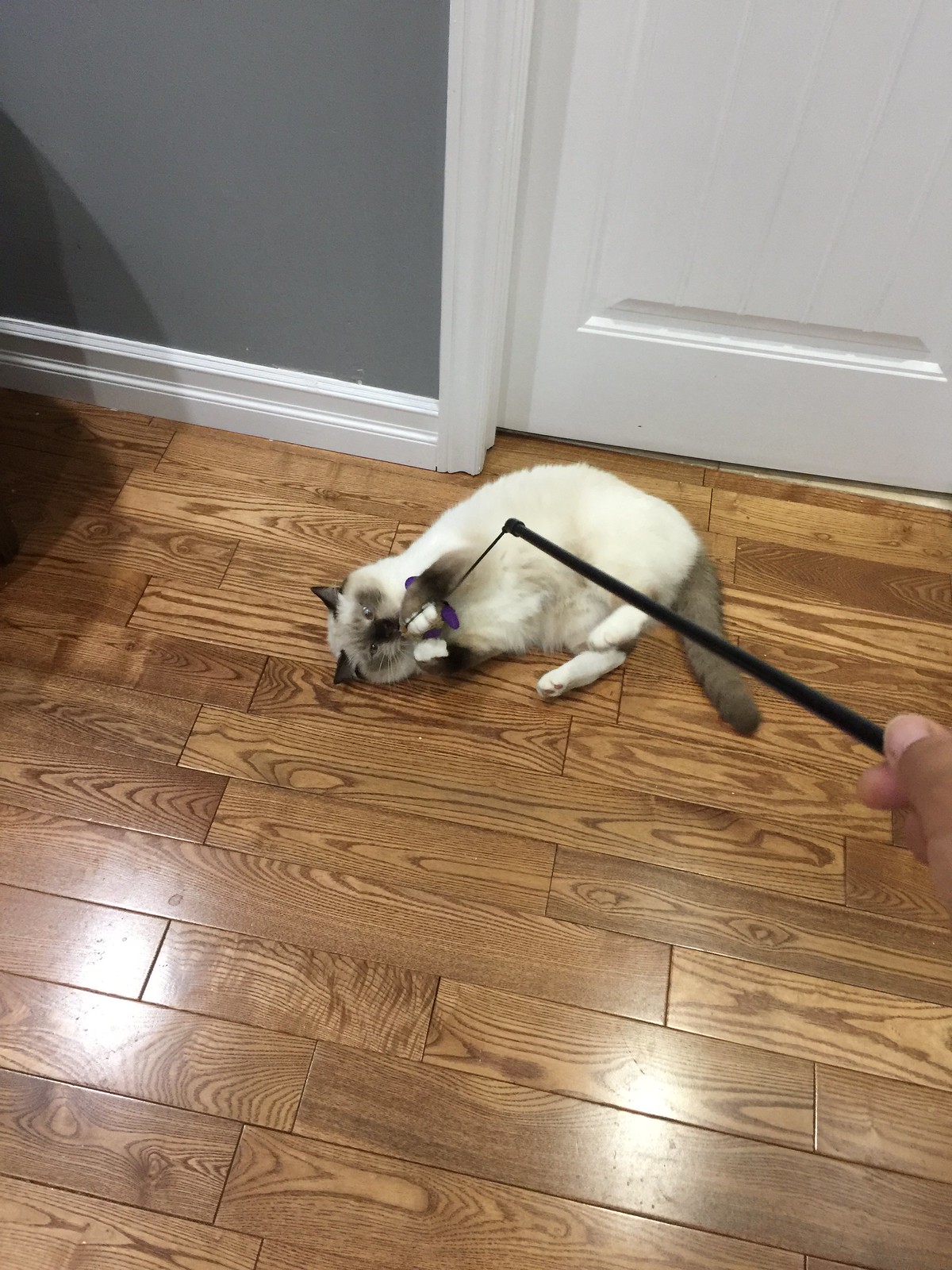In this picture, a white cat with gray ears, a gray tail, gray front legs, and gray patches around its eyes is lying contentedly on its back on a shiny, clean wooden floor. The floor, made up of brown wooden planks, features distinct wood grain swirls and lines, and has a few spots where light reflects off its surface. Behind the cat is a white door with a door frame, next to a medium gray painted wall. To the right side of the image, a hand with four visible fingers holds a black plastic wand, dangling a purple toy—possibly a bird or a butterfly—on a string. The cat has the toy gripped firmly in its front paws, which are white at the tips, and appears to be enjoying playing with it.